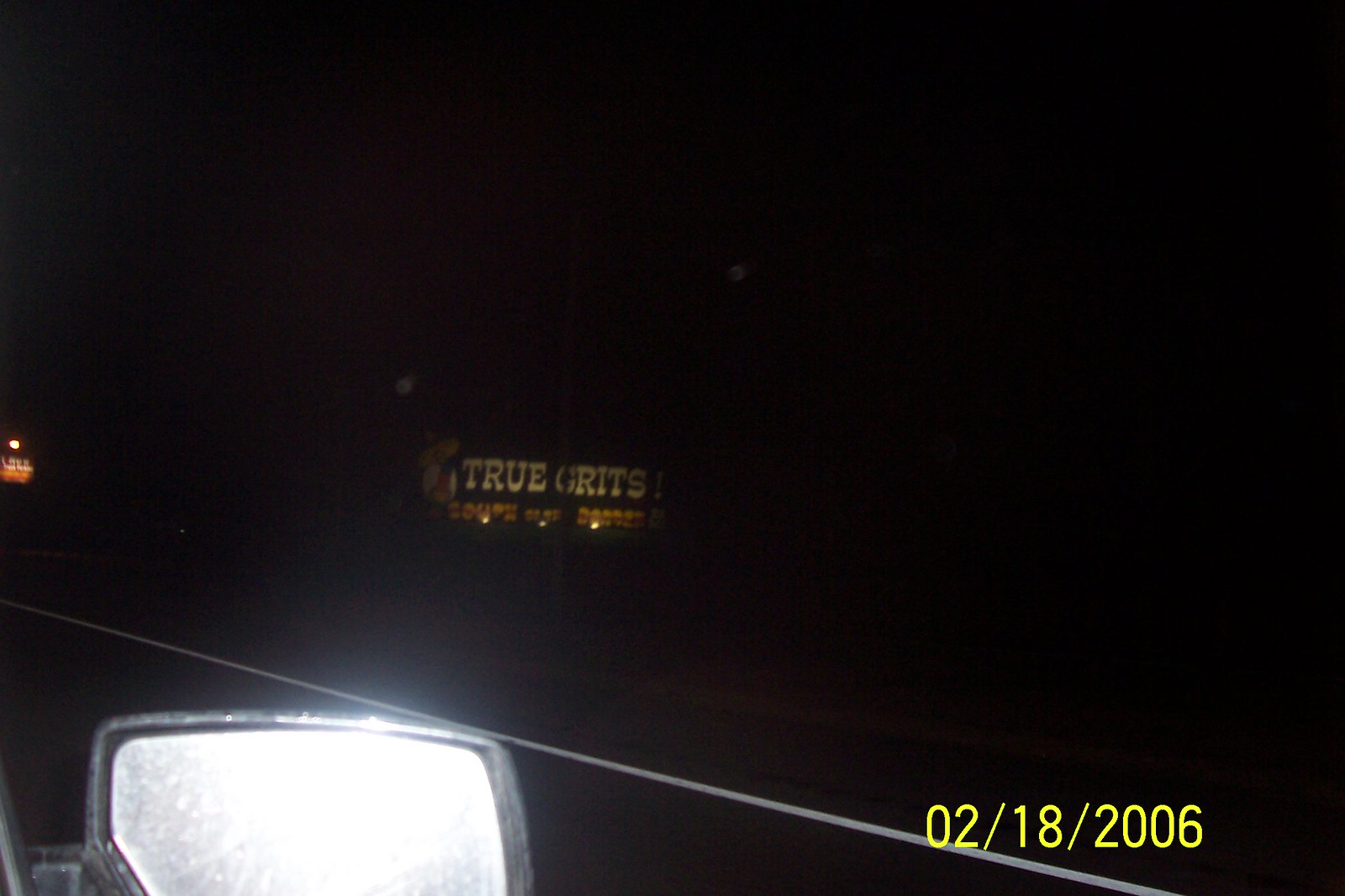The photograph captures a nighttime scene from the perspective of a passenger in a car. The backdrop is mostly black, indicative of a dark night sky, with a hint of an orange glow off in the distance. Cutting diagonally across the bottom of the image, there's a white line marking the edge of the road. In the bottom left corner, a side mirror with a black frame brightly reflects light from the camera. Dominating the center of the image is a distant billboard with the text "True Grits" in white against a dark green background, illuminated by three small solar lights beneath it. Below this, there is additional orange text, though it is too blurry to be legible. On the right-hand side, yellow text displays the date "02-18-2006." Another barely visible sign can be seen far off to the left, adding to the depth of the scene. Overall, the photograph encapsulates the serene and somewhat eerie ambiance of a nighttime drive.